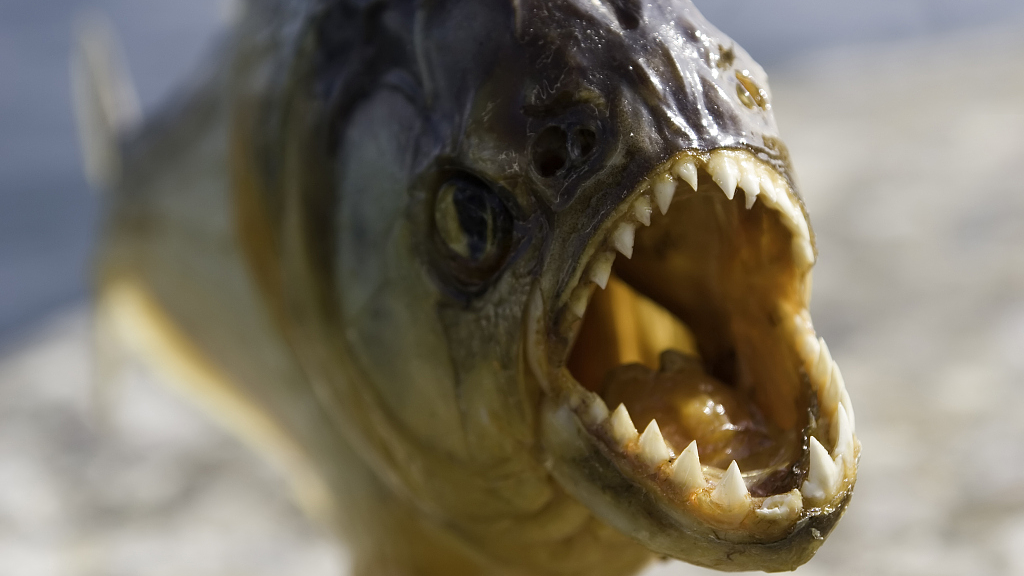The photograph is a startling, up-close image of a piranha fish, primarily focusing on its gaping, wide-open mouth filled with numerous razor-sharp, white teeth. The inside of the piranha's mouth is large and hollow, displaying a yellowish-tan hue. The terrifying, fang-lined mouth is front and center, drawing immediate attention. The fish is mostly shown from the front view, with its brown-yellowish face and nostril holes clearly visible. Its yellow eye with a vertical black pupil adds to its menacing appearance. The lower part of the piranha's body is a dull yellow, transitioning to a darker brownish color towards the top, which nearly appears black. The background is blurred with areas of white and blue, keeping the focus squarely on the piranha's formidable mouth and sinister gaze.